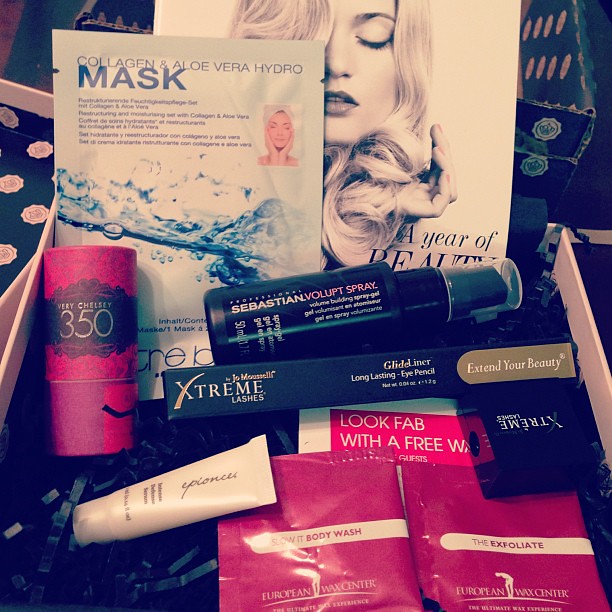In the picture, there are several beauty products meticulously laid out, with a prominent image in the background showcasing a blonde woman with her eyes closed and one hand near her face, exuding a seductive vibe. The text on this backdrop reads "A Year of Beauty." Among the products, the "Collagen and Aloe Vera Hydro Mask" stands out, featuring splashes of water and a woman's face with her hands framing her chin. Also present are items in red plastic wrapping labeled as body wash and exfoliate, branded with "European Wax Center." Black containers hold various creams, and there is a cylindrical "Sebastian Volupte Spray" along with a product labeled "Very Cherry 350." Additionally, an item for "Extreme Lashes" is included. The color scheme of the packaging varies, with notable black and pink tones, indicating a diverse array of bath, body, and hair care products.